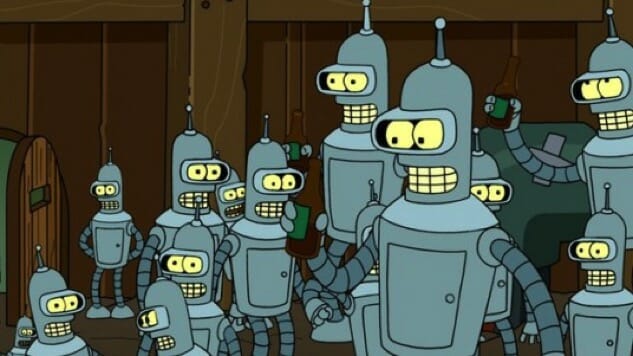This image is a detailed cartoon scene featuring a group of silver robots resembling characters from the show Futurama. There are about eleven of these robots, each sporting two creamish white eyes and a smile of three rows of teeth. They have a distinct design with an antenna on their heads topped with a white ball and torso that looks almost like a can with striped arms. Most noticeable, some of the robots on the right side are holding brown beer bottles with green labels, seemingly in the midst of a toast. In the background, there's a wooden wall and an arched wooden door on the far left side of the picture, adding to the setting that might resemble a factory or workshop. The overall composition of the image is rectangular.